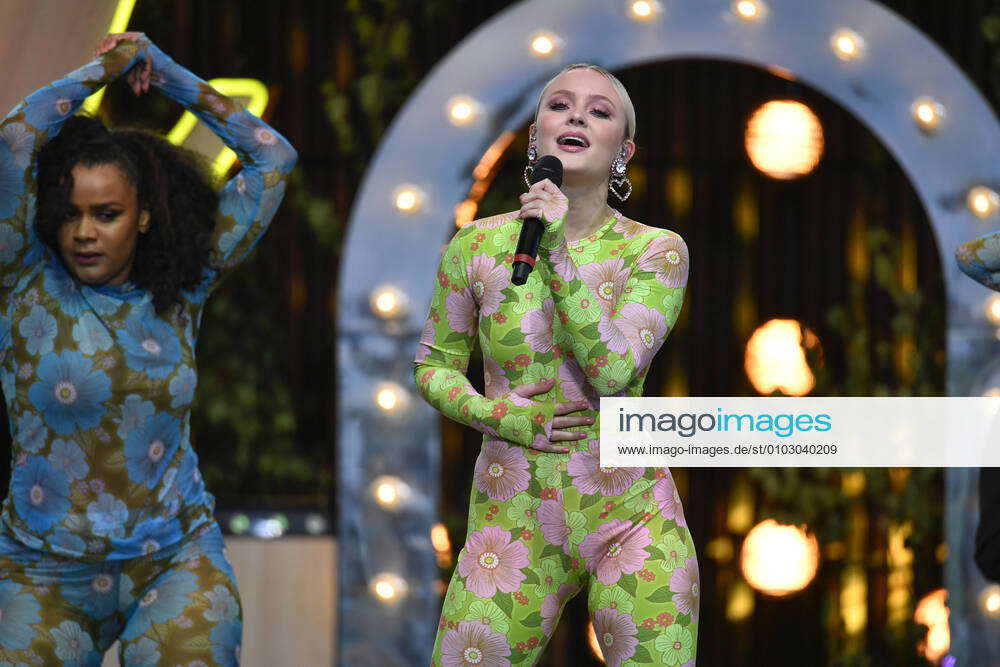In this detailed photograph, two performers are captured in the midst of their act. The performer on the right, center in the image, is a light-skinned, blonde-haired woman adorned in a bodysuit featuring a pattern of green leaves and pink flowers. She is holding a microphone up to her mouth with her left hand, seemingly in the middle of singing, her mouth open, with her other hand positioned in front of her waist. She is accessorized with diamond heart-shaped earrings and wears noticeable makeup.

To her left is another performer, a dark-skinned woman with bushy hair cascading around her shoulders. She is dressed in a bodysuit with a black and dark blue floral pattern, characterized by dark blue poppy flowers. Her arms are raised above her head, suggesting she is dancing.

The backdrop includes an arrangement of floodlights and an illuminated upside-down horseshoe-shaped arch with three vertical lines hanging from it. In the lower right corner of the image, a white rectangular band prominently displays the text "Imago Images." The word "Imago" is in black or dark gray letters while "Images" is in blue. Beneath it, the website www.imago-images.de followed by additional characters can be discerned.